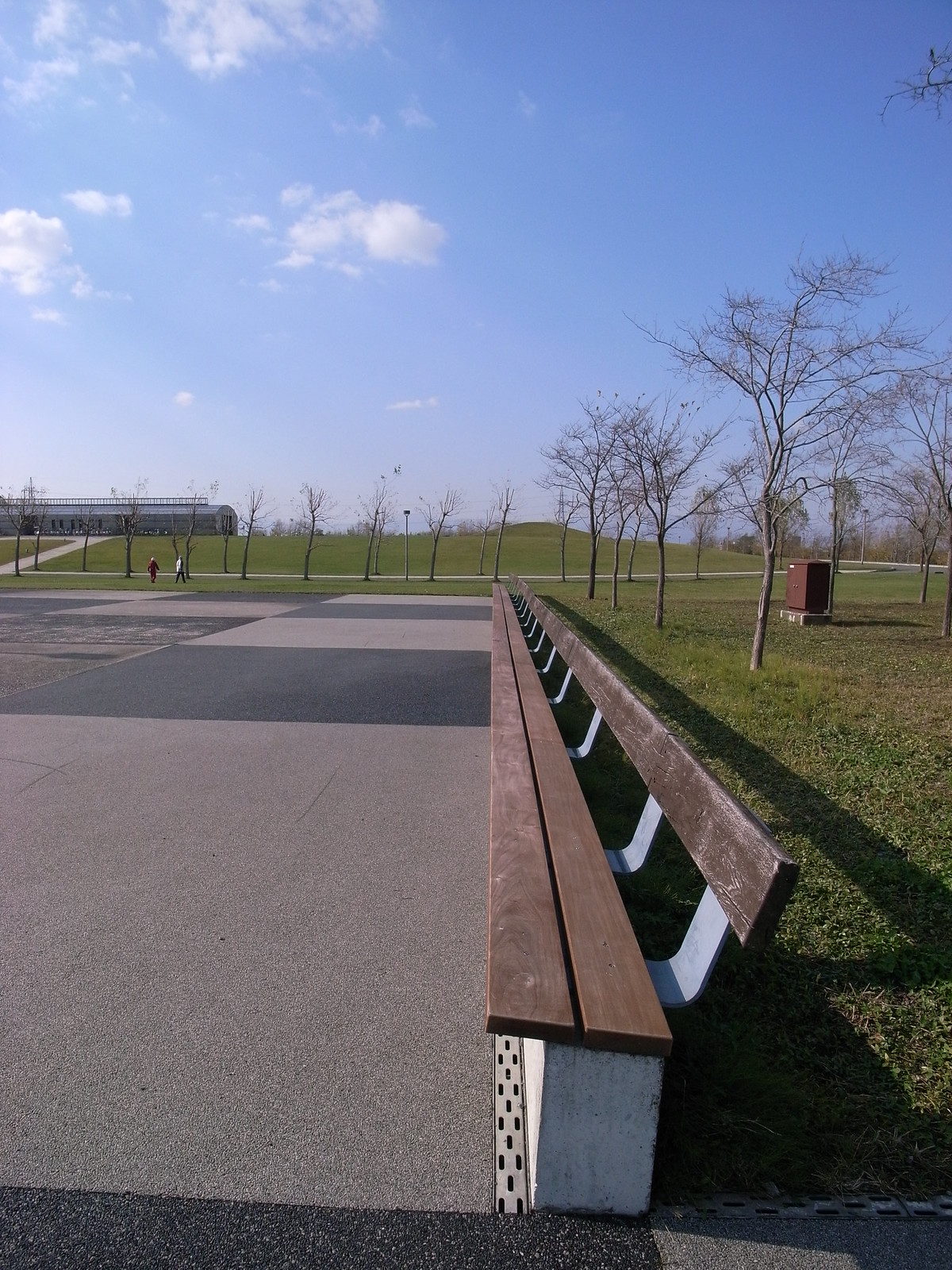This photograph captures a meticulously composed scene at an outdoor park on a sunny day. The sky is a gradient of blue, adorned with a few white, wispy clouds, particularly clustered on the left side. The long, central focus of the image is an extensive wooden bench that stretches impressively across a large, checkered concrete area. The bench, built with two wooden planks for the seat and a single wooden plank for the backrest, is supported by metal bars and casts a shadow on the grass behind it, indicative of the sunlight coming from the top left.

Directly behind the bench is a small grassy area populated with several young trees that have shed their leaves, suggesting it's either fall or early spring. Further back in the image, there's a pathway that meanders through the grass and connects to a large, gray building. This building, on the left edge of the photograph, has a visible sidewalk leading out from its front. Additionally, the image captures two figures in the distance, one dressed in red and the other in white, contributing to the lively yet serene atmosphere of the park. The entire scene suggests a newly developed public or recreational space, perhaps a recent addition to an urban development or a newly built community area.